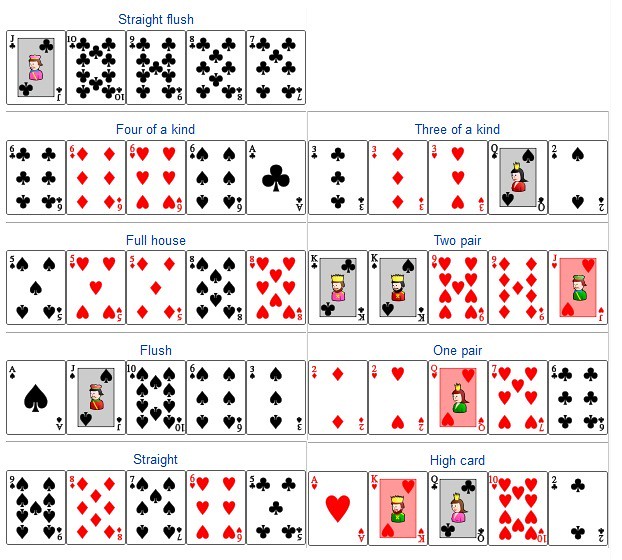The image is an informative chart illustrating various poker hands using playing cards, with a square layout where all sides are equal in length. The chart features five rows displaying different poker hands, with the bottom four rows containing two sets of hands each, and the top row featuring one set.

At the very top of the chart, there is blue text that reads "Straight Flush." This hand consists of a Jack of Clubs, a Ten of Clubs, a Nine of Clubs, an Eight of Clubs, and a Seven of Clubs. 

In the second row, the left hand is labeled "Four of a Kind" in blue text. It displays a Six of Clubs, a Six of Diamonds, a Six of Hearts, a Six of Spades, and an Ace of Clubs. The right hand in the same row is labeled "Three of a Kind" in blue text and shows a Three of Clubs, a Three of Diamonds, a Three of Hearts, a Queen of Spades, and a Two of Spades.

The third row starts with a hand labeled "Full House" in blue text. This hand consists of a Five of Spades, a Five of Hearts, a Five of Diamonds, an Eight of Spades, and an Eight of Hearts. 

This detailed chart provides a clear visual guide to understanding different poker hands, showcasing each hand with accompanying labels for ease of learning.